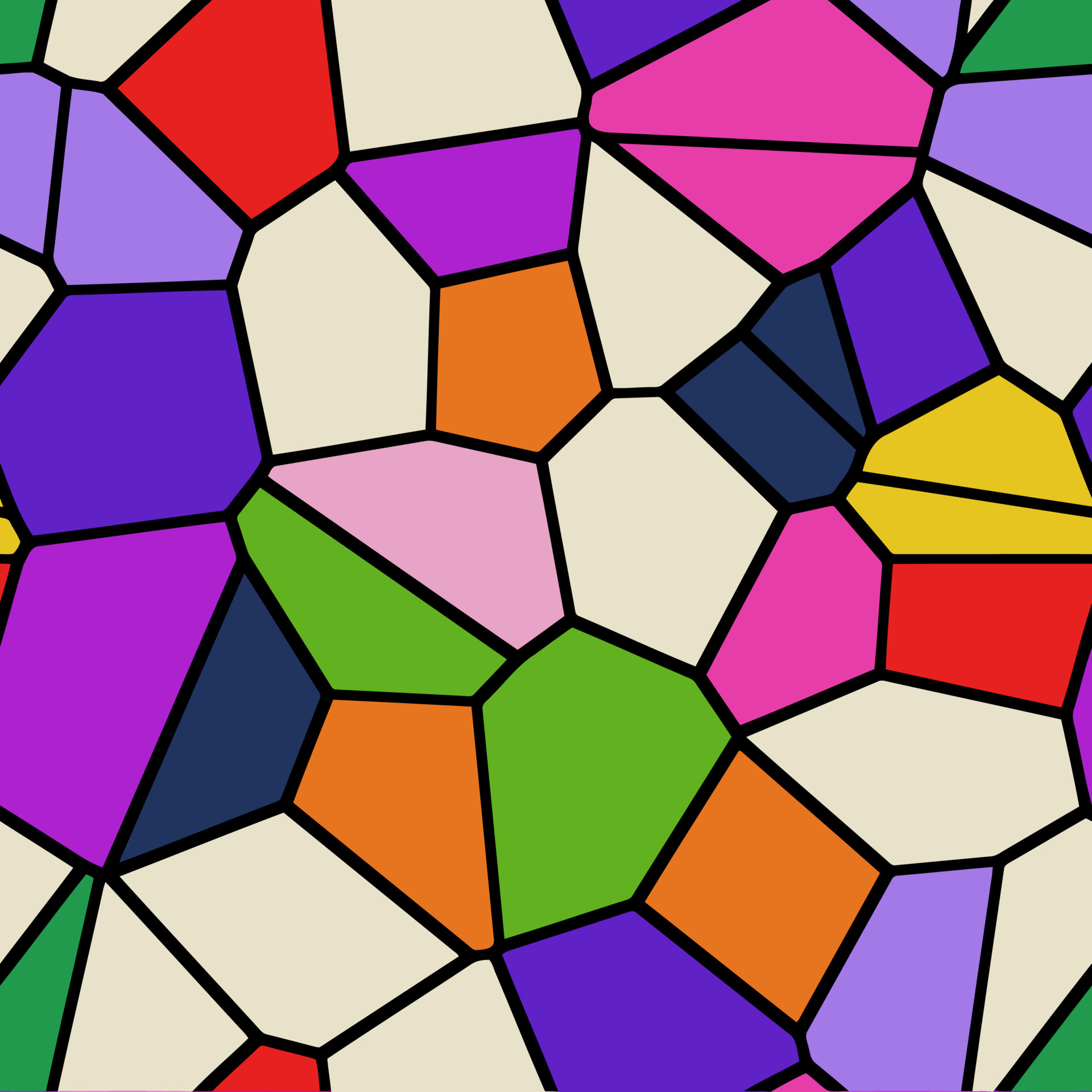The image is a highly detailed drawing that evokes the appearance of stained glass, filled with an intricate arrangement of thin black lines forming a variety of geometrical shapes. These shapes include hexagons, pentagons, squares, and irregular polygons, all tightly interlocked without any gaps. Each shape is filled with a different bright and vibrant color, creating a jumbled yet harmonious visual spectacle. The colors range from lime green, kelly green, and varying shades of blue, to multiple hues of purple, pink, red, orange, yellow, and cream. The dominant cream color, along with the assortment of magenta, navy, dark blue, and fuchsia, add to the piece’s complexity. The entire image maintains a consistent square shape and gives off a simplistic yet dynamic impression, reminiscent of a colorful mural or constellation.